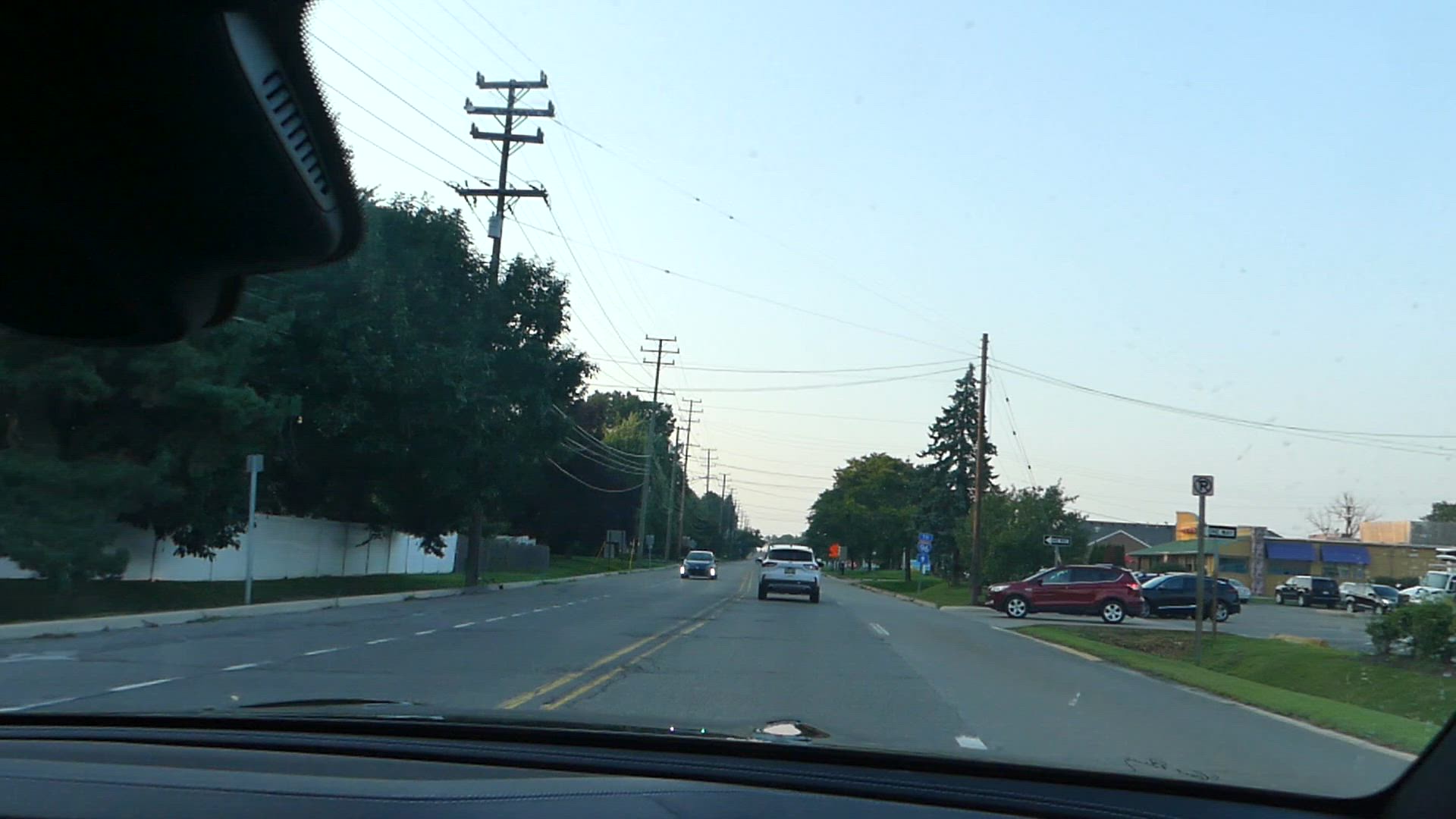The image, captured from within a car via a dash cam, prominently features the car's hood at the bottom. The top left corner of the photo shows the vehicle's middle console, positioned against the upper portion of the windshield. The scene reveals a two-lane road, where the car is traveling in the left-hand lane. 

Directly ahead, a blue Prius is approaching, positioned a few hundred yards away. Further up the road, a restaurant is visible, with a red sedan attempting to pull out from the parking area and a red SUV preparing to make a right turn. Additional parked cars, including a couple of black vehicles, can be seen near the restaurant.

Both sides of the road are lined with trees, radiating lush greenery. The left side is marked by telephone poles and a classic white picket fence, adding a touch of quaint charm to the roadside scenery.